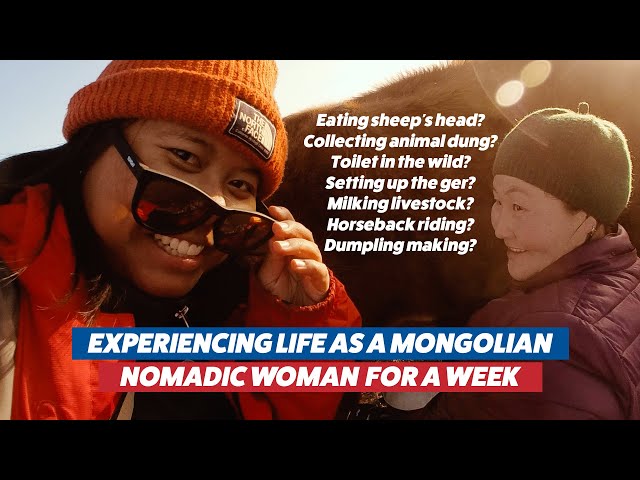In the advertisement, two women are featured prominently against a sunlit backdrop, suggesting an outdoor setting. The woman on the left is smiling directly at the viewer, wearing a North Face orange beanie and an orange jacket. She is pulling down her sunglasses to reveal her eyes. To her right stands an older indigenous woman dressed in a brown or green hat and possibly a warmer, purple-toned jacket. She is smiling as she looks at the other woman. Between them, bold white writing lists adventurous activities: “Eating sheep's head, collecting animal dung, toilet in the wild, setting up the gear, milking livestock, horseback riding, dumpling making.” At the bottom of the image, the text reads, “Experiencing life as a Mongolian nomadic woman for a week,” emphasizing the cultural and immersive experience. There appears to be a hint of a horse's mane, adding to the nomadic theme. The sunlight filters from the top right, enhancing the warm and inviting feel of the advertisement.